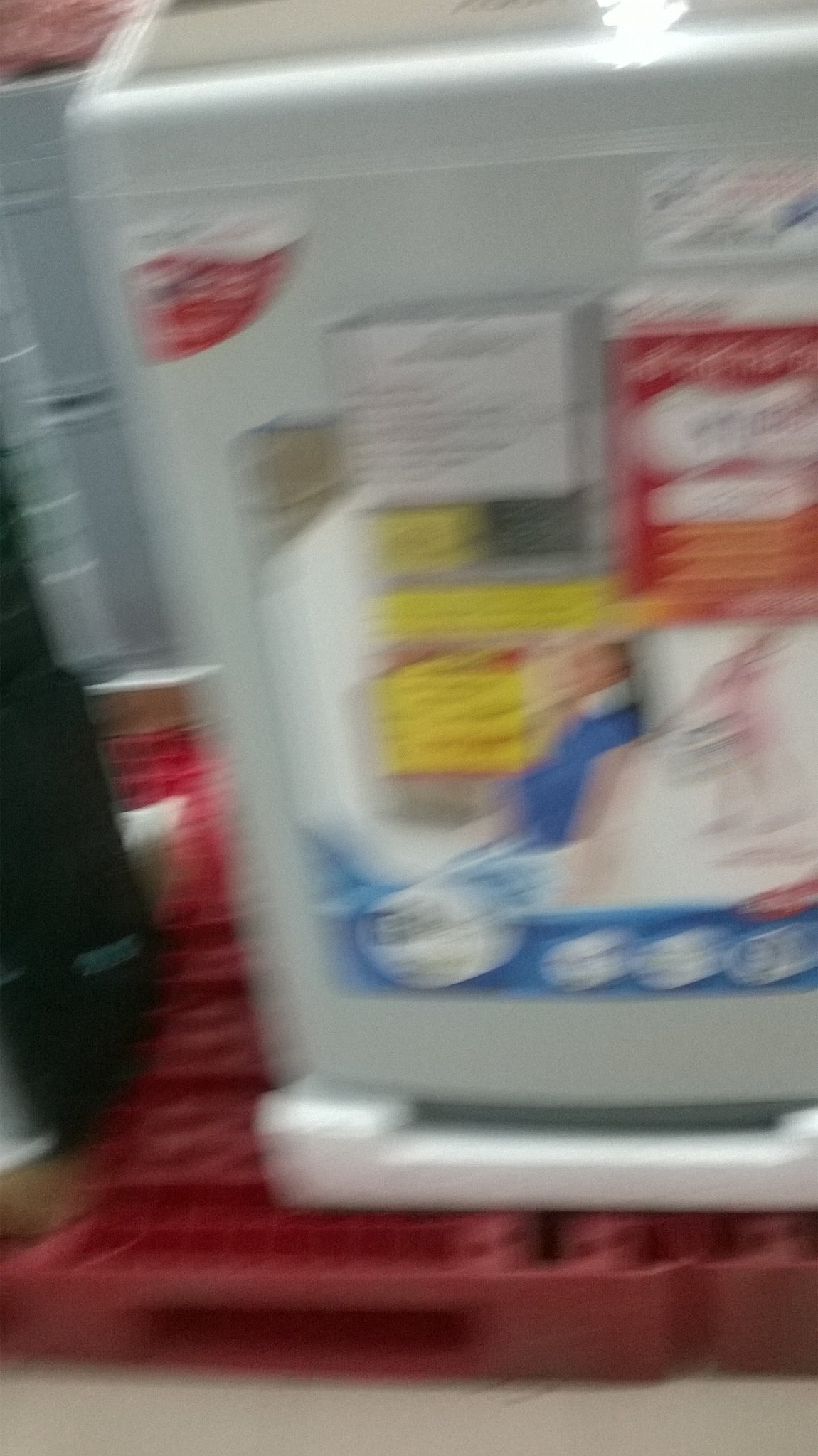The photograph captures a blurry image of a top-loading white washing machine with rounded edges, standing on a red plastic pallet and a base of white foam. The washing machine is adorned with multiple white, red, and blue stickers with unreadable text due to the blurriness. The background, imbued with a grainy texture, suggests a retail environment, likely a store selling white goods appliances. Additional appliances can be seen displayed on the same red plastic pallet. Adjacent to the washing machine, there’s a black object whose details are indistinguishable in the unclear image. Hues of pale yellow, teal blue, and light brown are also present, adding to the diverse but indistinguishable color palette of the photo.